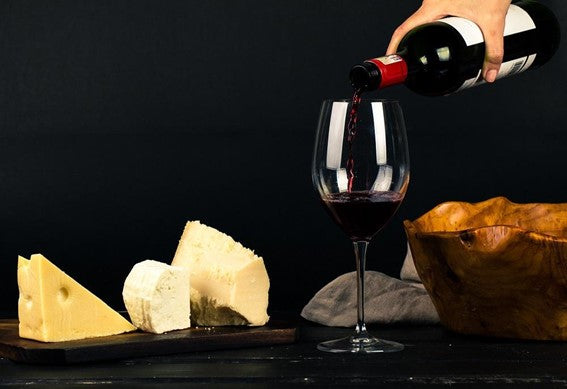In this captivating photograph, a white male is seen pouring dark red wine into a typical wine glass, with his hand visible at the top right of the frame. The background is an all-encompassing black, creating a striking contrast to the scene. Below, the wine and cheese rest on a black, wooden table, adding to the sophisticated ambiance. To the left of the man, an array of cheeses is displayed: a hard cheddar cheese, a creamy Brie cheese in the middle, and a soft yellow cheese to the right. The cheeses are presented in various shapes, some sliced into triangles and others haphazardly cut. Further to the right of the pouring wine, there is a wooden bowl and a basket with unseen contents. Behind the wine glass, a gray cloth drapes subtly to the left, complementing the setting. This well-staged image evokes a sense of indulgence, perhaps hinting at a cozy night in with fine wine and eclectic cheeses.